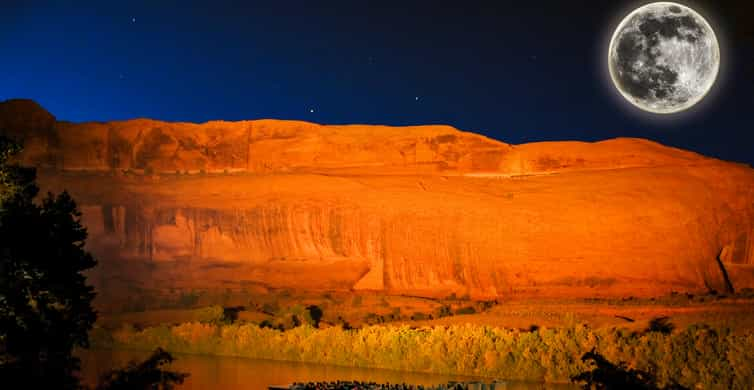This nighttime color photograph captures a striking scene of a canyon in the southwestern United States, reminiscent of the Grand Canyon. Central to the image is a large, irregularly shaped cliff, glowing in hues of red and orange, bathed in light from an artificial source emanating from the upper left. At the base of the cliff runs a river, reflecting the illuminated cliffside and surrounded by lush trees and shrubbery. The sky above is a deep, dark blue, dotted with a few visible stars. Dominating the upper right-hand corner is the moon, depicted in shades of white and black, adding a dramatic touch to the serene landscape. This unique photograph exquisitely blends natural beauty with the eerie glow of artificial light, highlighting the canyon's vibrant colors against the peaceful night sky.